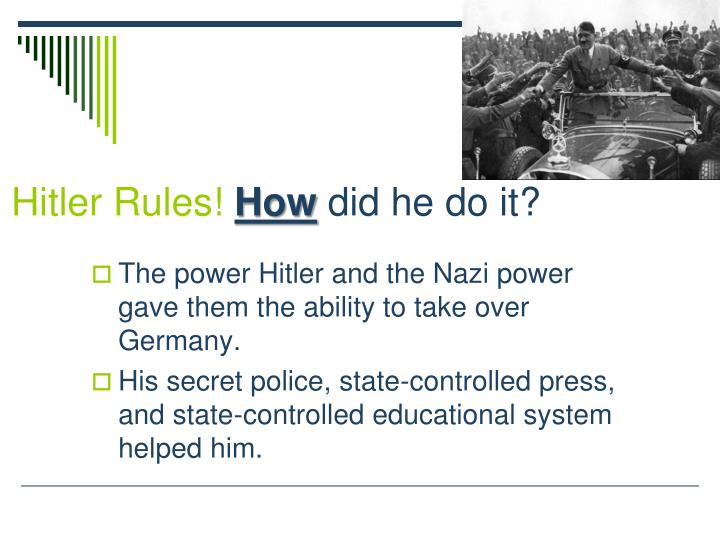This image is a PowerPoint slide from a history class with a detailed infographic. The background is plain white, and the slide features a logo in the upper left corner consisting of green-striped triangles. At the top is a horizontal line. On the top right, there is a black-and-white photograph of Adolf Hitler standing in a Mercedes-Benz convertible. He has his arms stretched out, shaking hands with the crowd that surrounds and cheers for him, with many people reaching out towards him.

The main text of the slide reads "Hitler rules!" followed by "How did he do it?" with "how" underlined and in bold. There are two bullet points beneath this title: "The power Hitler and the Nazi power gave them the ability to take over Germany," and "His secret police, state-controlled press, and state-controlled educational system helped him." The layout is simple, with the bulk of the slide dedicated to text and the photo, and minimal additional graphic elements.